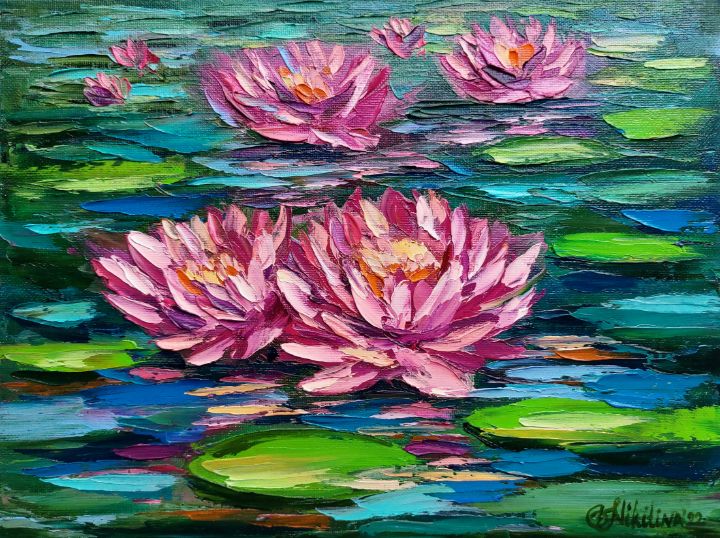The painting depicted in the image is an oil on canvas creation inspired by the style of Monet, showcasing a serene pond scene. Predominantly filled with green lily pads, the composition leaves only small patches of blue water visible. The central focus is on the blooming water lilies, featuring thick pink petals and vibrant centers of orange and yellow. The arrangement includes two larger flowers surrounded by three smaller ones at the top, and two additional prominent blossoms near the bottom middle. The layers of paint are visibly textured, revealing the artist's technique. The artist's signature, located on the bottom right, suggests the work was completed in 2022.